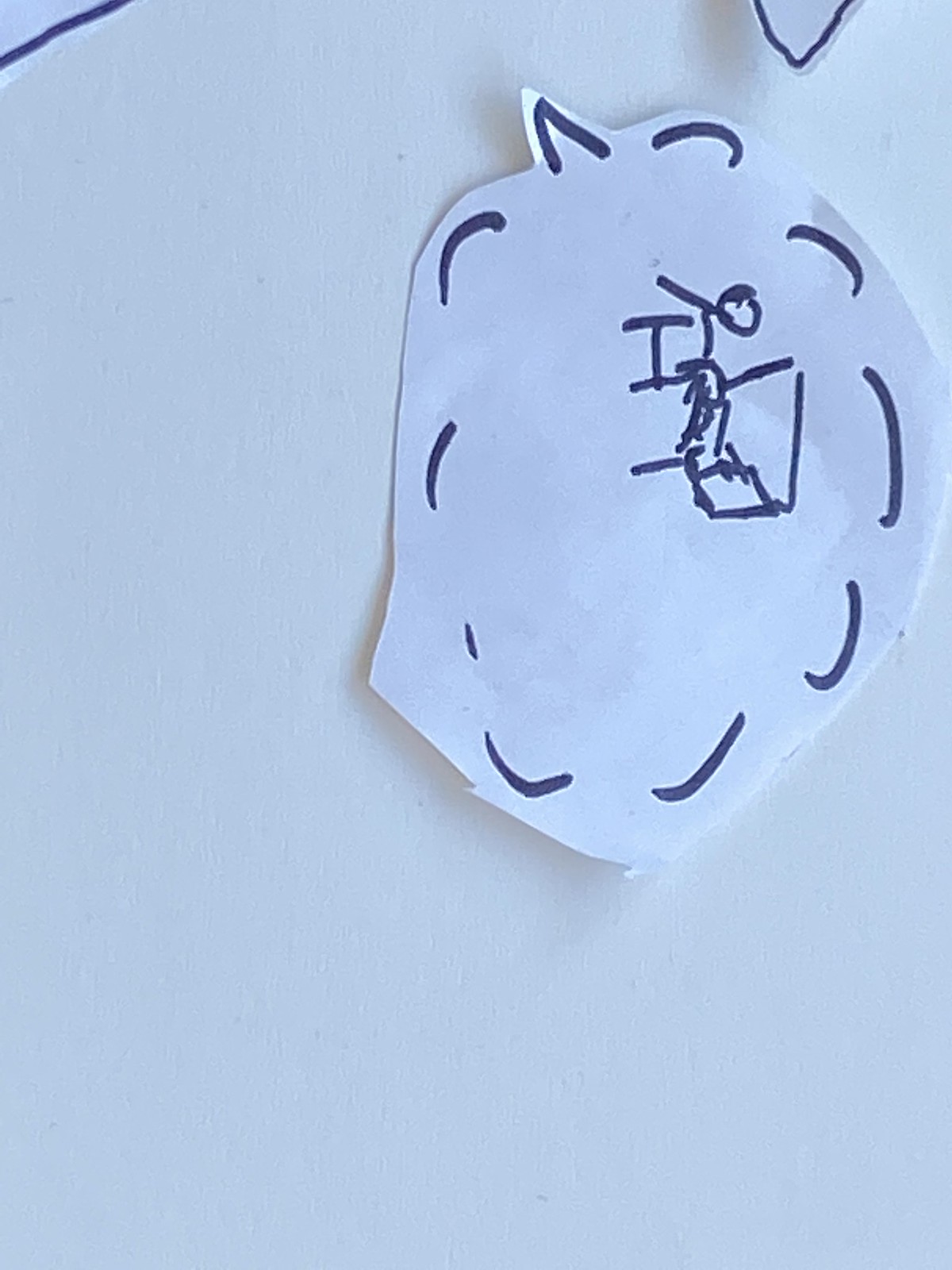The image features an unevenly cut piece of paper shaped like an oval, positioned on a white background that resembles a whiteboard. The oval paper’s edges are jagged and sharp. In the top left corner of the image, a grainy area displays a thick, dark black line running diagonally. The upper right corner reveals a smaller triangular piece of paper marked with what looks like a black letter 'V'. This triangular piece also rests on the white background and seems to be slightly elevated, casting a faint shadow underneath.

Along the sides of the oval paper, from the 12 o'clock to the 11 o'clock position, there are small, curved lines that resemble eyebrow shapes. Just to the left of the top curved line is an upside-down black 'V' on a pointed edge of the paper, also appearing slightly raised due to the visible shadow beneath it.

In the center of the oval paper, there is a rudimentary, black stick figure resembling the letter 'H'. This figure is crude and simplistic, giving it a childish, scribbly appearance with minimal detail.